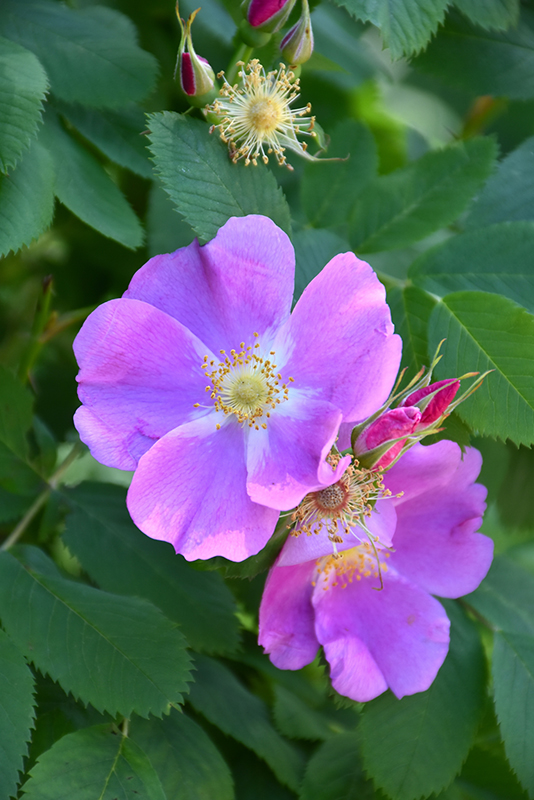This close-up photograph captures a vibrant outdoor scene featuring two prominently purple flowers situated in the middle of a dense patch of tiny, jagged green leaves on light green stems. The rectangular image, with its vertical side being much longer than the horizontal, highlights the striking details of the flowers and surrounding foliage. Positioned centrally are the two fully bloomed flowers with light purple petals and a distinctive light yellow center, surrounded by darker yellow buds tipped with minute yellow balls, likely pollen. To the right of the main flower, only half of a similar flower is visible, appearing slightly darker due to the play of shadows. Nestled between the two main flowers are two unopened buds, red in color, hinting at future blooms. The clarity of the image, enhanced by bright natural daylight, provides a vivid and detailed view of this floral arrangement. The bright setting and clear details make this image a captivating display of nature's intricate beauty.